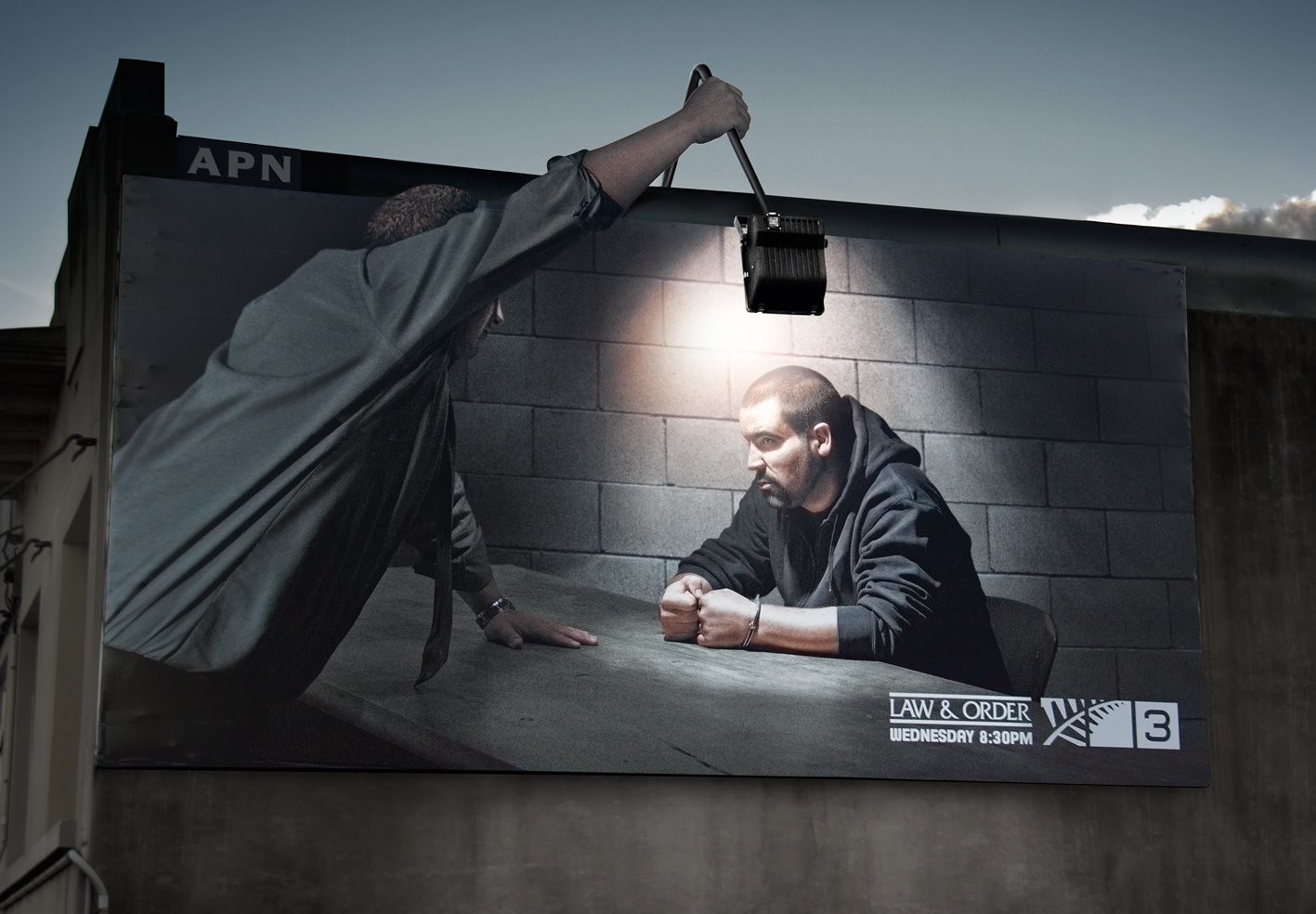This image features a striking billboard on the side of a building adorned with the letters "APN" near its roof. At the very top of the picture, a sliver of sky with barely discernible clouds is visible. The billboard promotes the TV show "Law and Order," announcing new episodes airing at 8:30 PM on Wednesdays. Accompanying this text are a symbol and the number "3," likely indicating the local channel broadcasting the show.

The central image on the billboard depicts a tense, dramatic scene typical of the show, where a police detective interrogates a handcuffed suspect. A compelling optical illusion is created by an exterior light mounted on the building. This light, though fixed in place, appears in the context of the billboard as if the detective is holding it, casting a focused beam directly onto the suspect.